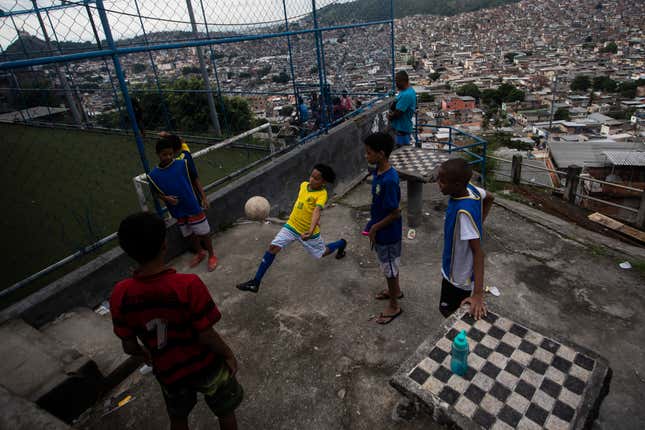The image captures a vibrant scene right outside a caged soccer arena, set on a dirty cement pad atop a cliff in a village overlooking a bustling, dilapidated city. Seven children are featured prominently in the foreground, actively engaged in a game of soccer or keep-up with a dirty white ball. The children are dressed in a mix of colorful soccer jerseys and blue pinnies, implying team play. One boy, sporting a Brazil shirt, is among those in action, while another leans against a concrete chessboard etched into a built-in table with a blue bottle on top. To their left, the fenced soccer field stands as a backdrop, creating a contained area with two goals and space for belongings. In the far background, the city sprawls densely with weathered buildings under overcast skies, framed by distant mountains. A few adults linger in the background, adding to the lively atmosphere of this communal playing area.